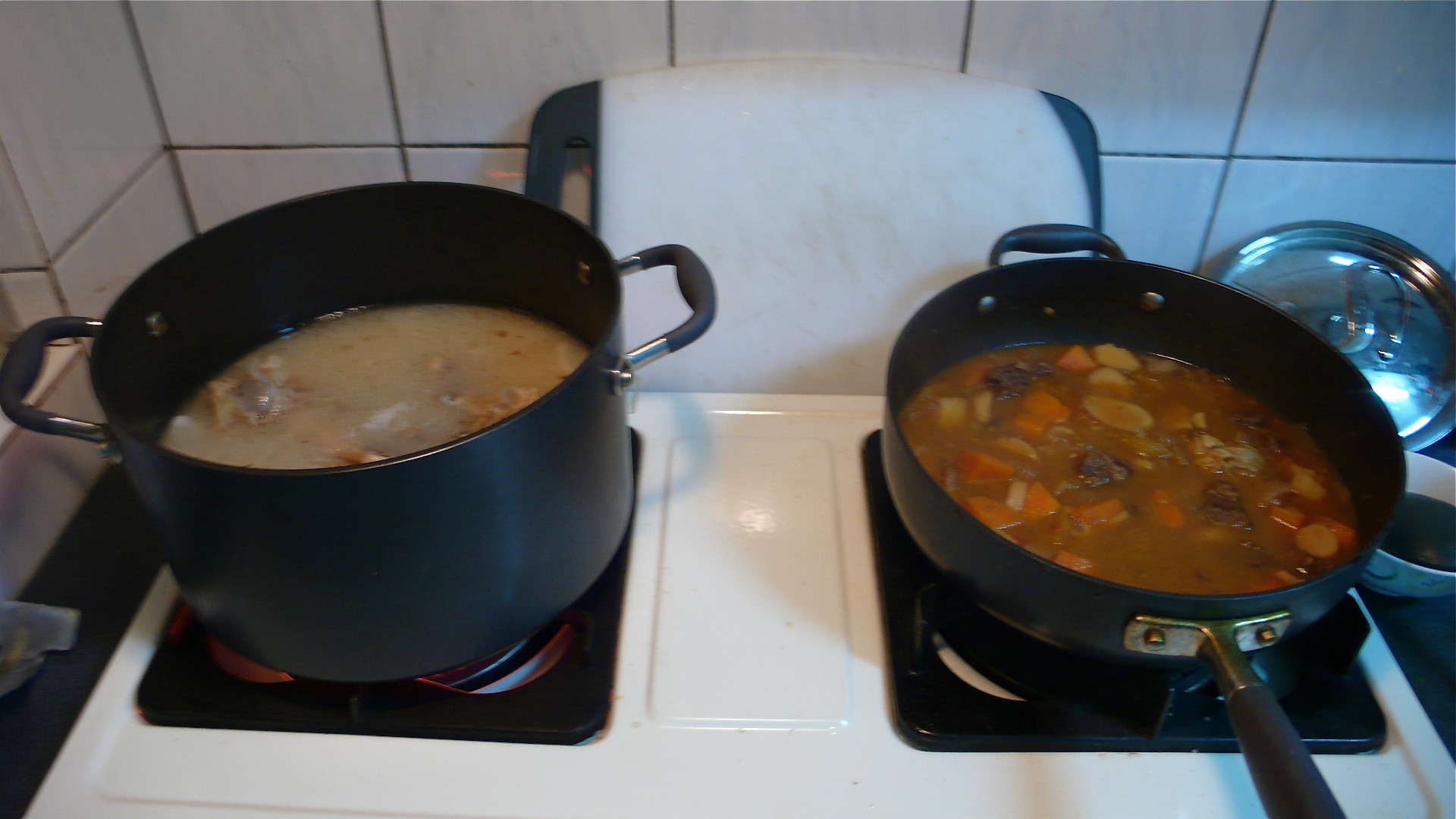In this detailed photograph, a clean white stove with two square burners takes center stage. The left burner supports a dark greyish pot filled with a yellowish soup, likely chicken, while the right burner holds a stir fry pan with a grey handle, containing a hearty brown stew with visible chunks of beef, potatoes, and carrots, similar to a curry. Both containers are detailed with visible metal bolts on the handles. Adjacent to the burners, a silver pan cover rests on the countertop. The stove features a white lip that separates the burners. Behind the stove, off-white tiles with grey grout provide a subdued backdrop, with a grey chair draped with a white towel partially visible. Additionally, mounted on the back of the stove against the tiles is a white plastic cutting board with black handles.